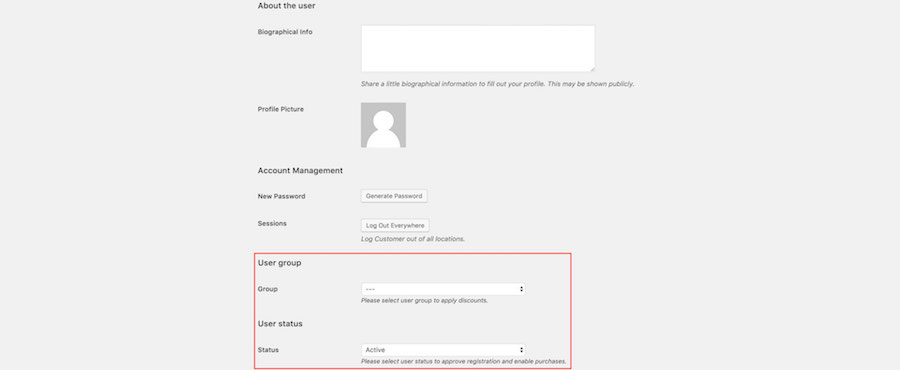The background of the image is predominantly a large, light gray square. At the top, there is very small black text with the heading "About the User." Below this heading is the segment titled "Biographical Information," where biographical details about the user are to be filled in. To the right of this section, there's a white rectangle approximately five inches long and three inches high, underneath which it prompts, "Share a little biographical information to fill out your profile. This may be shown publicly," in very small black text.

Positioned below this text on the left side of the image is the placeholder for the profile picture. This is represented by a gray square containing a simple white outline icon of a person, depicting a circle for the head and broader shapes for the shoulders and body.

As you move further down, the "Account Management" section appears. Below this, there is a field to input a new password with a button to the right labeled "Generate Password" inside a box. Continuing downward, there is a section labeled "Sessions" to the right of which is the option "Log Out Everywhere." Just beneath this, there is a description indicating "Log out of the account on all locations."

At the bottom-right corner of the image, there is another set of options within a red-outlined square. The inside of this square is gray, with choices labeled "User Group," "Group," "User Status," and "Status." Beside this section, there is a smaller box containing the word "Active."